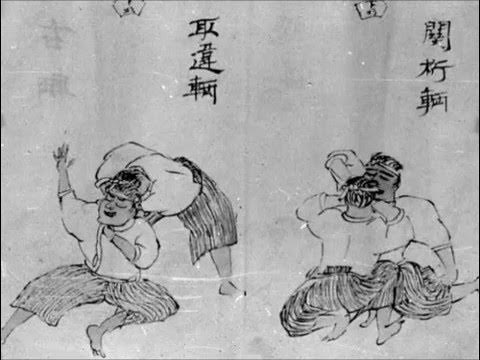This black and white Japanese-style illustration, reminiscent of ancient Asian artwork, depicts scenes of wrestlers against a textured, faded paper background. On the lower left side, two men are engaged in combat; one man sits on the floor with his right arm outstretched, wearing a white shirt and striped pants, while another man, whose head is obscured behind the seated wrestler, arches his back dramatically. On the lower right side, the same two men now face each other closely, both barefoot and wearing white headbands, white shirts, and striped pants. Their intimate positioning suggests a moment of connection or pause in their wrestling. Above both sets of wrestlers, Asian characters are inscribed, adding to the traditional feel of the scene. The overall composition is rendered with what appears to be a fine black pen or marker, contributing to its detailed and aged appearance.